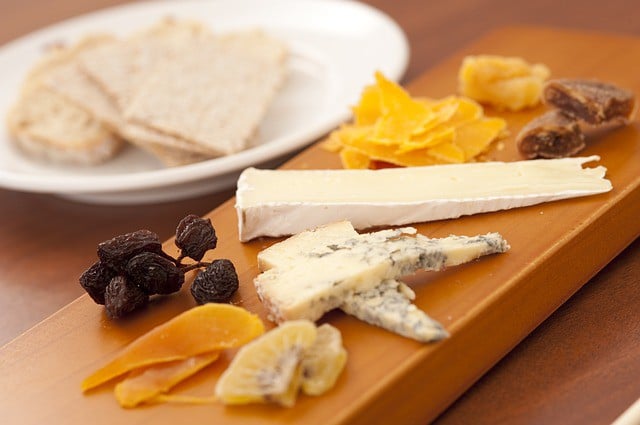In this detailed image, an orange-lacquered board stretches diagonally from the bottom left to the top right, showcasing an array of gourmet delights. The centerpiece is an assortment of cheeses, including a distinct blue cheese and a creamy triangular white cheese. Surrounding the cheeses are various edibles: possible candied fruit, shriveled berries that could be dates or raisins, and other orangey-yellow items that might be dried ginger or similar delicacies. Positioned in the background on a darker laminate tabletop is a blurred white bowl filled with rustic crackers, complementing the cheese board. The overall setting appears to be indoors, perhaps in a cheese shop, with no visible text to identify the items. The scene is a harmonious blend of brown, white, orange, and dark blue tones, with the in-focus cheeses drawing the eye to the center of the composition.